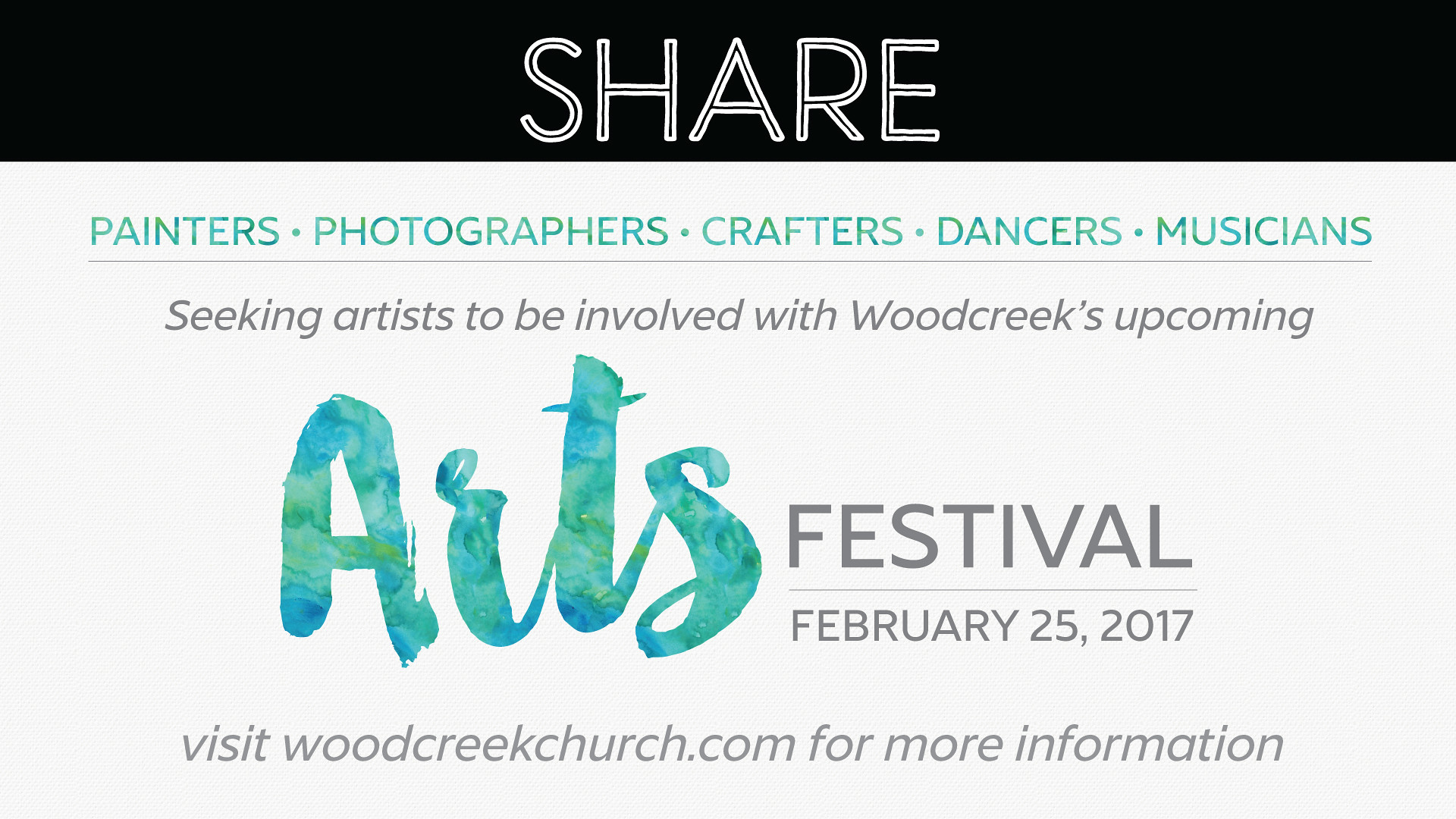The image appears to be a rectangular advertisement, possibly for a festival or event, set in a horizontal orientation. At the top, there's a thin black banner with the word "SHARE" prominently displayed in white, all capital letters, and centered. Below this banner, the background turns white, featuring the words "Painters," "Photographers," "Crafters," "Dancers," and "Musicians" in a teal green font, each word separated by a small dot. Further down, in black text, it reads: "Seeking artists to be involved with Woodcreek's upcoming," leading to a larger, calligraphy-styled word "ARTS" in a watercolor effect, blending blue and green hues. The word "FESTIVAL" follows in all capital letters and a gray font. The event date is given: "February 25th, 2017," and the advertisement concludes with a call to action in gray text: "Visit woodcreekchurch.com for more information."